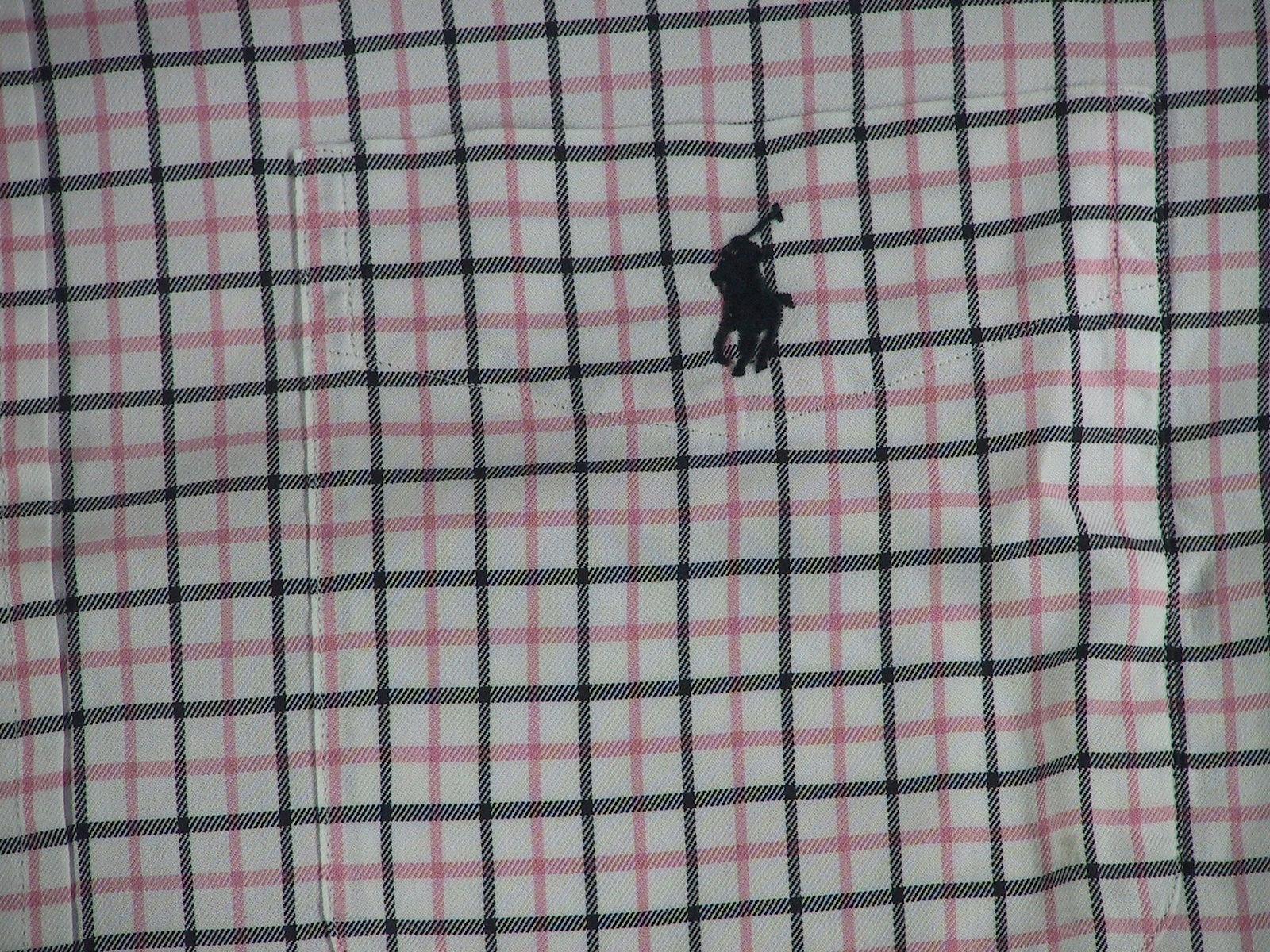This color photograph features an extreme close-up view of the fabric from what appears to be the front pocket of a shirt. The fabric has a light gray background adorned with a windowpane plaid pattern. The plaid design is composed of darker gray and light pink lines, creating a subtle yet intricate grid-like effect. Prominently displayed on the pocket is a designer logo, which is a black silhouette of a horse. Although the exact brand is not identifiable, the detail and texture of the fabric are vividly captured, highlighting the shirt's sophisticated design.